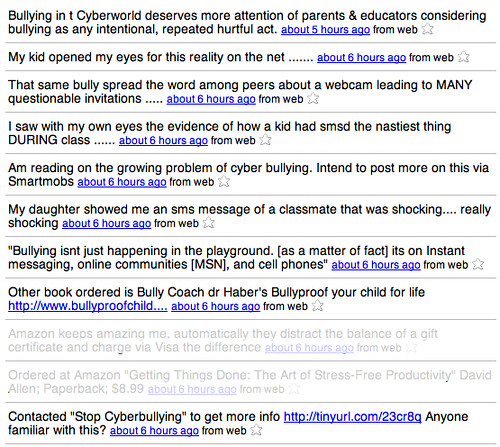The image depicts a screenshot of what appears to be a forum or a website focusing on various instances and discussions around cyberbullying. The content displays a series of headlines or the first lines of posts, each linking to more in-depth discussions. One post reads, "Bullying in the cyber world deserves more attention of parents and educators, considering bullying as an intentional, repeated, hurtful act," followed by a timestamp of approximately five hours ago. Another headline shares a personal story: "My kid opened my eyes to the reality on the net," marked as six hours ago. Further down, a troubling report is highlighted: "That same bully spread the word among peers about a webcam, leading to many questionable invitations," also from six hours ago. Additional posts mention direct observations of harmful messages sent during class and emphasize the growing problem of cyberbullying, with timestamps generally around five to six hours ago. The entries suggest a continuous conversation and offer clickable links for more details. Toward the bottom, the image includes an invitation to "Contact Stop Cyberbullying to get more information," followed by a short URL. Some lower entries appear faded, indicating they might be less prominent or perhaps read. The overall impression is a stark visualization of ongoing, significant concerns over cyberbullying, aiming to provoke awareness and provide resources for help.